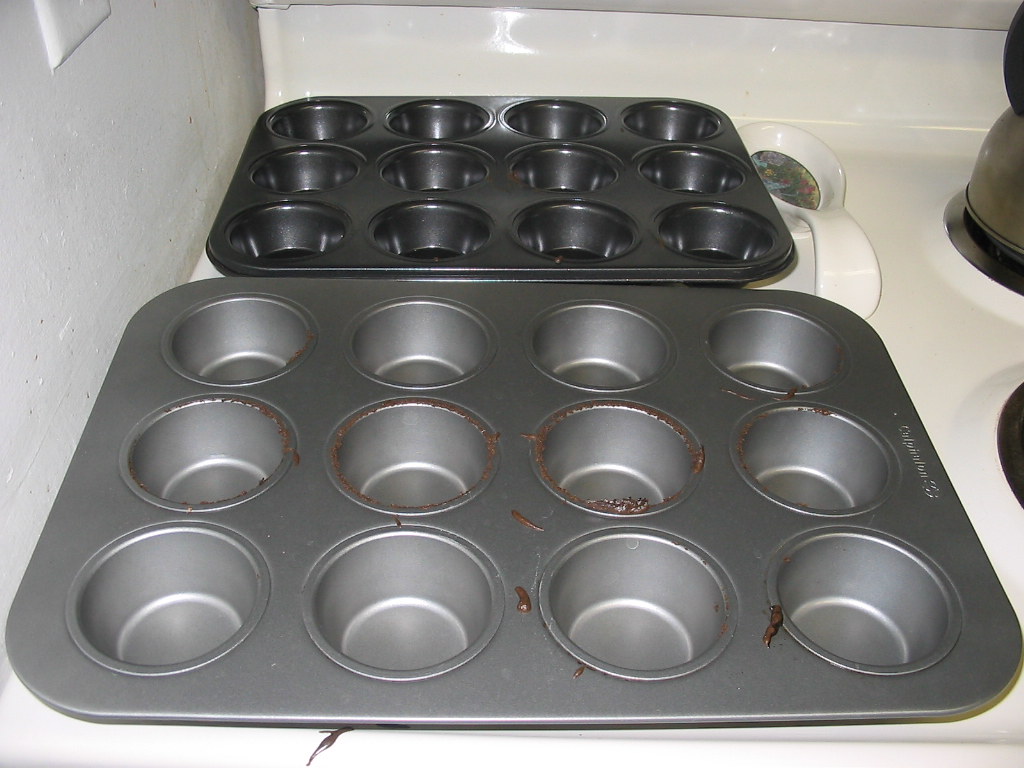The photograph captures a pair of well-used muffin pans, each with 12 slots, placed side by side on a white electric stove, revealing an array of kitchen details. The muffin pan in the foreground is a larger, silver chrome tray, evident by the visible chocolate residue around its rings and on the surface. The brand name is imprinted on the top right corner but is too small to read. The pan behind it is smaller, a metallic black color, and also bears traces of chocolate, suggesting it was used to bake the same type of muffins or cupcakes. To the right of the smaller pan, a white ceramic spoon rest with indistinct, colorful designs lies near the stove's rear burner, which holds a kettle. The photo also shows part of the front right burner and carries over the edges of the white, glossy kitchen surface and a partial view of a white wall on the left-hand side.